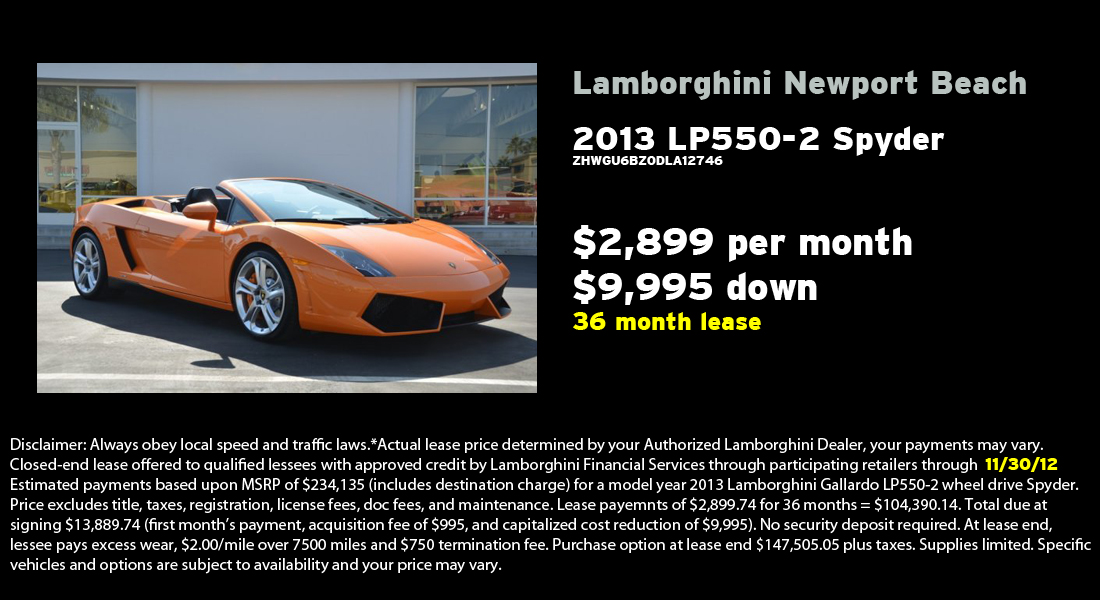The image features an advertisement for a Lamborghini dealership showcasing an orange 2013 Lamborghini LP 550-2 Spyder parked in front of a white building with large windows. The Lamborghini, with its top down, is set against a predominantly black background, making the vehicle stand out. On the right side of the image, details about the vehicle are provided, including the dealership name "Lamborghini Newport Beach," the model year "2013," and a specific code "ZHWGU6BCODLA12746." The pricing information states that the car is available for a lease at $2,199 per month, with a $9,995 down payment for a 36-month term. At the bottom of the image, there is a long disclaimer written in white font.